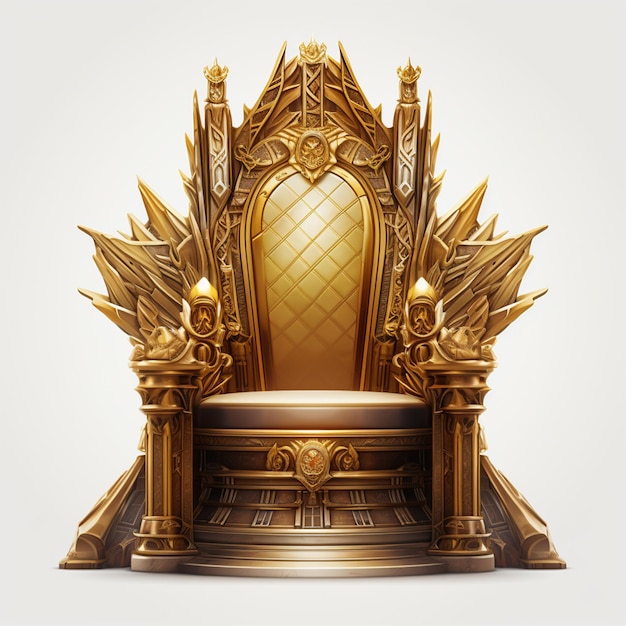This is a detailed, computer-rendered image of an enormous, fanciful throne, seemingly inspired by fantasy genres like Game of Thrones. The throne, designed for a king or a leader, showcases a highly intricate and elaborate design. Predominantly golden with hints of dark purplish-brown, especially at the base and lower part of the seat, the throne exudes an imposing and slightly sinister aura, reminiscent of a fantasy comic book style.

The high-arched back of the throne features a cross-hatched design, suggesting an overstuffed cushion for comfort. Both the seat and the backrest are cushioned, emphasizing luxury and opulence. Sharp, spike-like points emerge from either side of the seat, giving the impression of flames and adding to the dramatic appearance of the throne. The top of the throne also sports similar flame-like projections, further enhancing its majestic and powerful look.

The throne is elevated on a pedestal with columns and is rendered from a front point of view, making its grandeur fully visible. Additional ornamental details, including faces in the design, can be observed at the very top and just below the seat, showcasing an extraordinary level of craftsmanship and attention to detail.